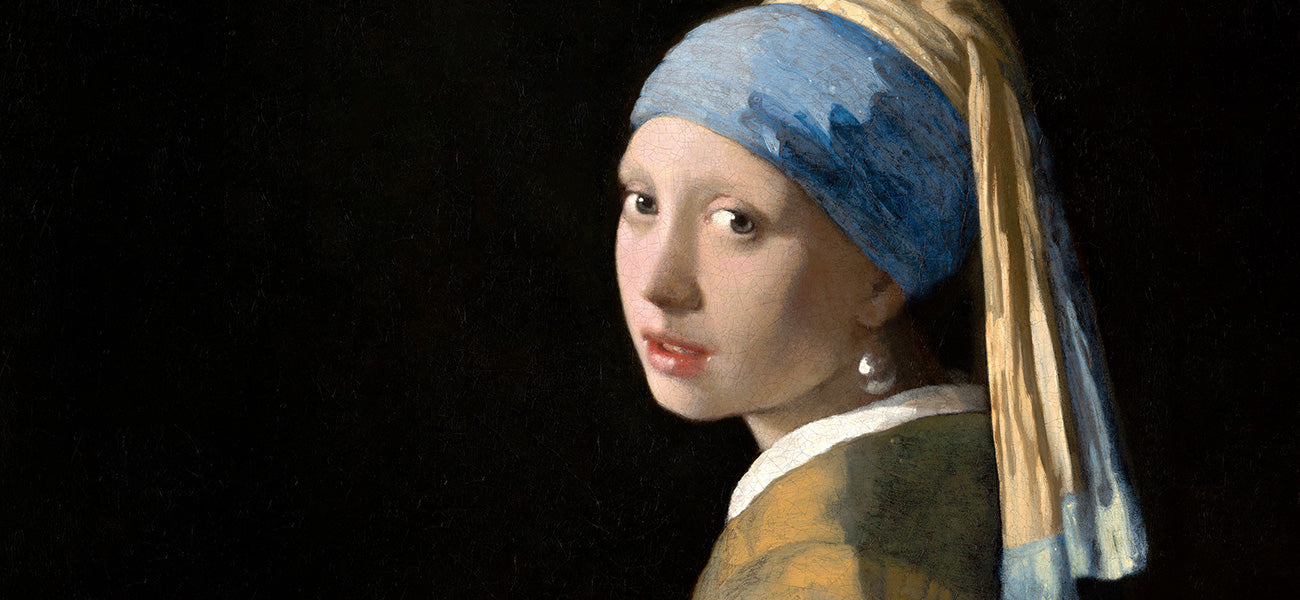The image is a captivating portrait of a young girl, photographed from the shoulders up, with a completely black background enhancing her presence. She is depicted in a side profile, glancing back with a curious expression in her bluish-brown eyes. Her hair is completely covered by an elaborate turban-like scarf that is blue where it touches her forehead and transitions to tan at the top, featuring two long, trailing ribbons—one brown and one blue with tassels.

She has a fair complexion, and her striking facial features include a beautiful nose, red lips adorned with lipstick, and a pair of circular silver earrings. Her attire consists of a white-collared garment with shades of green and possibly yellow hues. The portrait, with its horizontal and rectangular framing, emphasizes the girl's enigmatic yet inviting presence against the stark black backdrop.